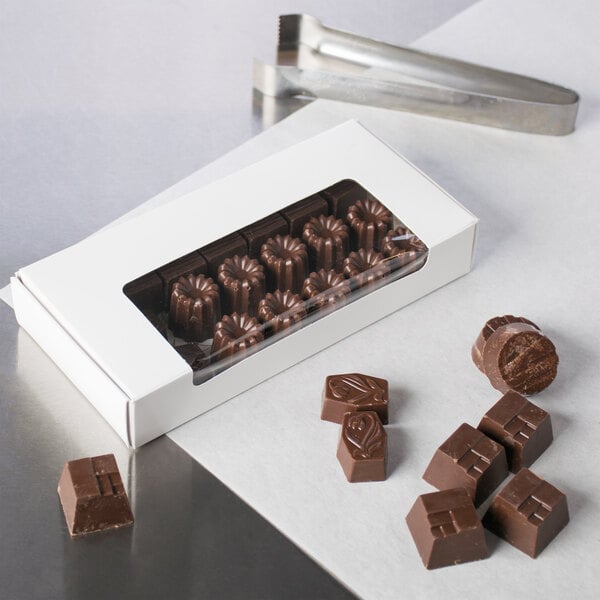This detailed photograph features an assortment of hand-crafted milk chocolate pieces displayed both inside a white box, with a plastic film cutout revealing the contents, and on a metal surface covered with white parchment paper. The chocolates, varying in shapes from cylindrical and flowery to flat-topped pyramid forms and hexagonal pieces, exhibit intricate designs pressed into their surfaces, including flowers and steps. There are around 10 chocolates inside the box, and an additional 8 or 9 scattered outside. Metal tongs, used for picking up the chocolates, are visible in the background. The overall scene is set against a predominantly white and silver color palette, with no text or additional elements to distract from the elegant presentation of the chocolates.